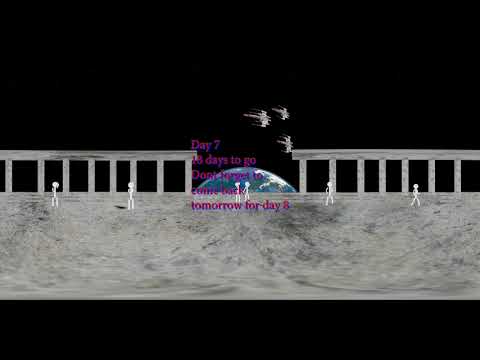The image appears to be a screenshot from a video game with a predominantly black background. Centered within this dark backdrop is a grey walkway, flanked by translucent barriers or railings, made of a material resembling white marble. Along this walkway, there are six clay-like model figures, spread out with two on the left side, two in the center, and two on the right. These figures have a simple design, consisting of basic head and body shapes without any clothing. 

In the middle of the walkway, extending into the backdrop, is a semi-circle resembling the top third of the Earth, set against the dark sky. Above this, three small spacecraft, reminiscent of X-Wing fighters from Star Wars, can be seen flying. Overlaying this scene, there is red text with the partially legible phrases: "Day 7," "13 days to go," and "Don't forget to come back tomorrow for Day 8." The text is somewhat obscured but stands out against the black and grey tones. The overall scene portrays a futuristic setting possibly indicative of a continuation or countdown within the game.